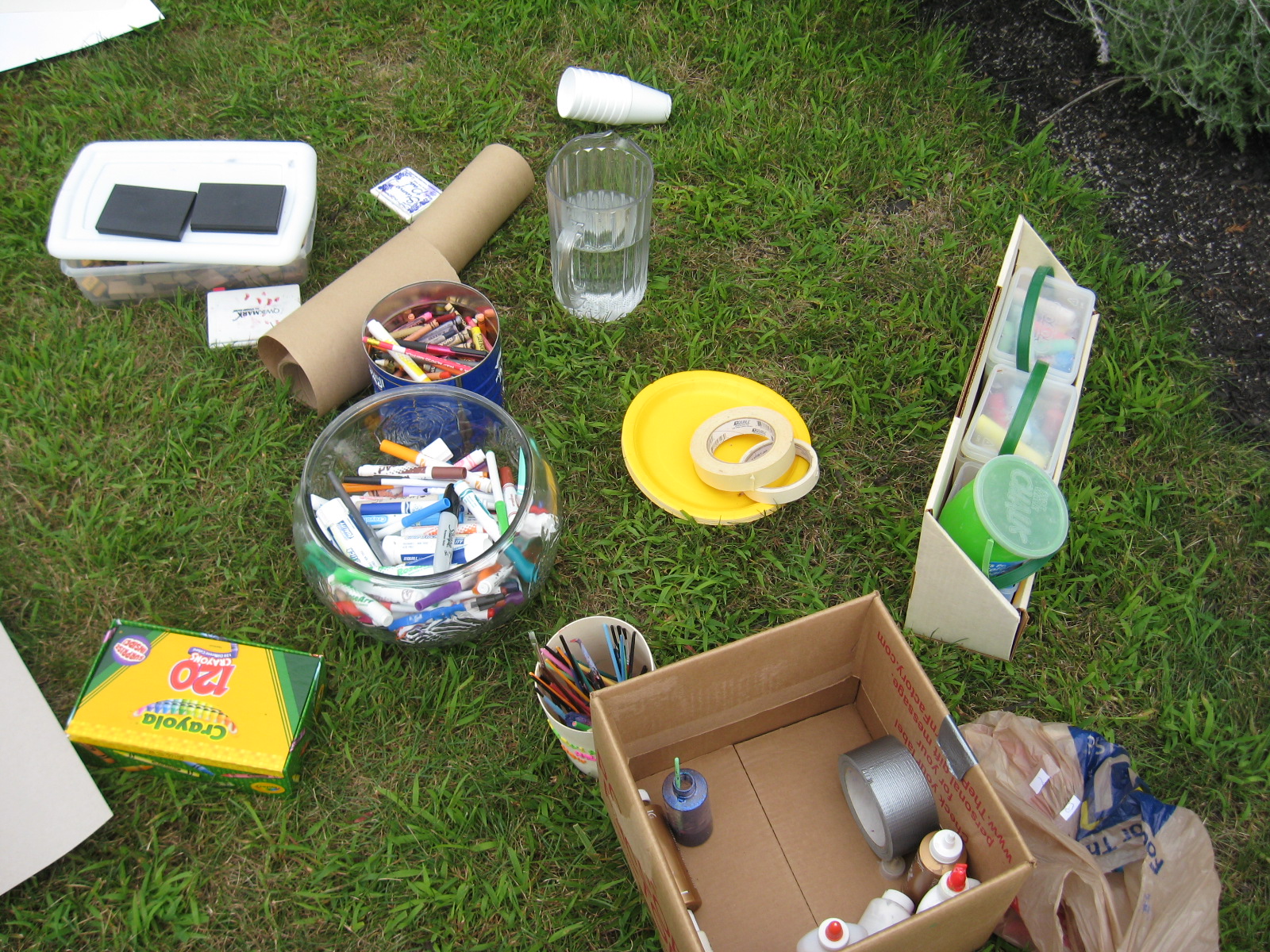A charming outdoor scene showcases a diverse array of art supplies scattered randomly across a vibrant green lawn. At the center of the slightly horizontal image sits a yellow plastic plate holding two rolls of masking tape. To the left of the plate, a fishbowl brimming with watercolor Sharpie pens stands about half full. Further left lies an upside-down box of 120 Crayola crayons, characterized by its iconic yellow and green design, accompanied by a single sheet of white paper positioned in the lower left-hand corner.

Continuing rightward from the fishbowl, one finds a plastic cup containing an assortment of small brushes—some with bristles pointing upwards, while most face down. Adjacent to this cup rests a medium-sized cardboard box with flaps folded inward, revealing an open bottle with an object extending above its cap on the left, a roll of silver tape on the right, and several bottles of Elmer's glue inside.

To the immediate right of this box, near the lower right-hand corner, lies a plastic grocery bag filled with unspecified objects. Above this, towards the right center, sits a cardboard container with angled sides, holding three tubs of rectangular opaque chalk. Between the container and the fishbowl, the yellow plate with masking tape reappears.

Directly above the fishbowl, a blue coffee can filled with crayons and pens is visible, with a sheet of craft brown paper located just above it. A large plastic tub with a white lid and clear bottom, containing what appears to be brown blocks or objects, occupies the upper center. Below this, a small cluster of white styrofoam cups accompanies a crystal glass pitcher, half-filled with water. The detailed arrangement of these art supplies creates a delightful tableau perfect for a creative outdoor session.